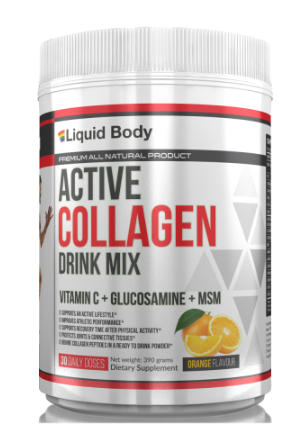This image features a product placement for the Activin Collagen Drink Mix by Liquid Body. The container is a large, full, gray bottle with a twist-off lid and a label that wraps entirely around it. The label predominantly displays the product name in black and red, stating "Active Collagen Drink Mix," followed by "Vitamin C + Glucosamine + MSM" components, suggesting its benefits for an active lifestyle. The flavor is clearly indicated as orange, with illustrations of orange slices and a green leaf adding a visual appeal on the bottom right. The label also highlights it as a premium, all-natural dietary supplement, suitable for 30 daily doses, with the net weight being 390 grams. The branding is accentuated with “Liquid Body” on the top left, accompanied by small rainbow icons, and a black line beneath it, underscoring the product’s high-quality image with the phrases "premium all-natural product." Little diamond designs add a touch of elegance to the overall presentation.